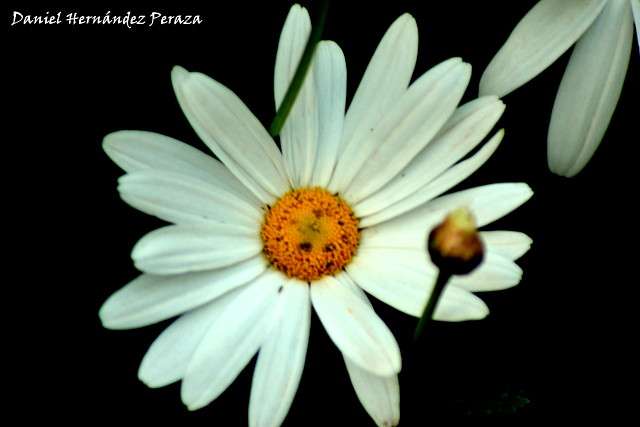This image showcases a beautiful white daisy flower with elongated, oval-shaped petals encircling a vibrant center that transitions from deep yellow to orange. The background is pitch black, rendering it almost invisible and providing a stark contrast that highlights the delicate details of the flower. In the upper left corner, the text "Daniel Hernandez Peraza" is written in white. There are several insects crawling around the central part of the flower, adding a touch of life to the scene. On the right side of the frame, a partially visible flower stem suggests a bloom that has already lost its petals. Additionally, the upper right of the image reveals three white petals from another similar flower, though the center is cut off by the frame. A green stem is draped over the topmost petals, adding texture and depth to the composition.